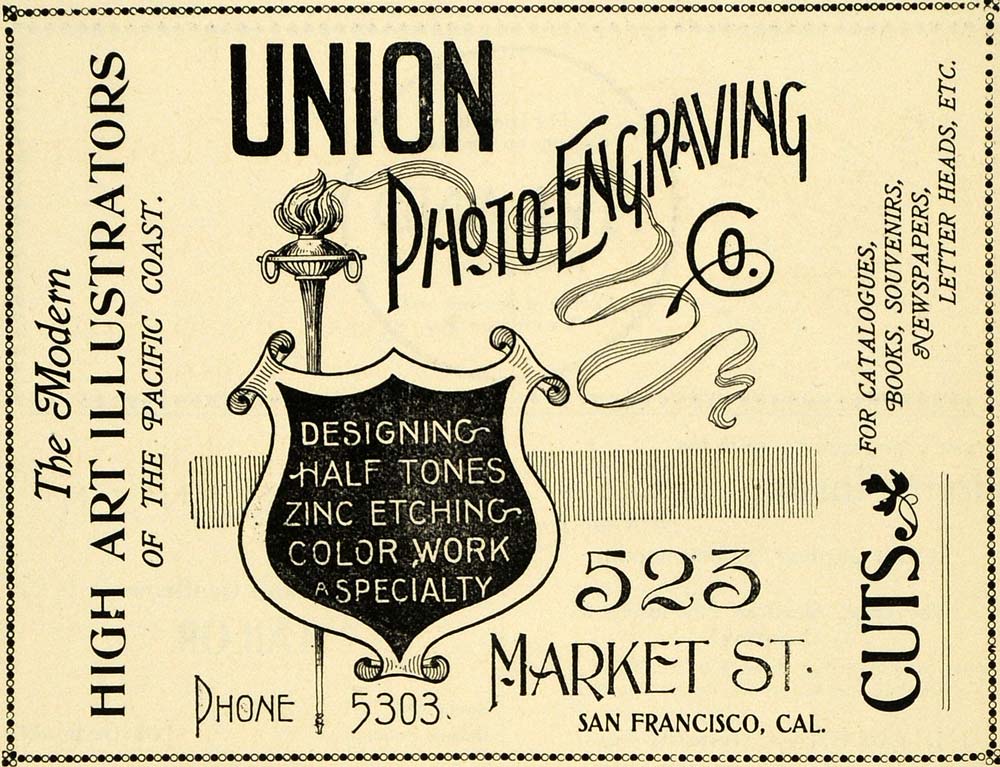The image showcases an aged advertisement with a cream-colored, slightly pinkish or light orange faded background, giving it an antique appearance. The ad is framed by a small border of alternating solid black dots and outlines of black dots. Prominently in the center, "Union Photo Engraving Co." is displayed in bold black lettering. Below this, there is an emblem featuring a torch and shield with white text on a black background that reads, "Designing Half Tones, Zinc Etching, Color Work a Specialty." Running vertically along the left side is the phrase, "The Modern High Art Illustrators of the Pacific Coast." At the bottom of the image, the address "523 Market Street, San Francisco, California" is provided along with a succinct phone number, "Phone 5303." On the right side of the ad, it lists services such as "Cuts for catalogs, books, souvenirs, newspapers, letterheads, etc." The overall layout features both vertically and horizontally oriented text, contributing to its vintage charm.